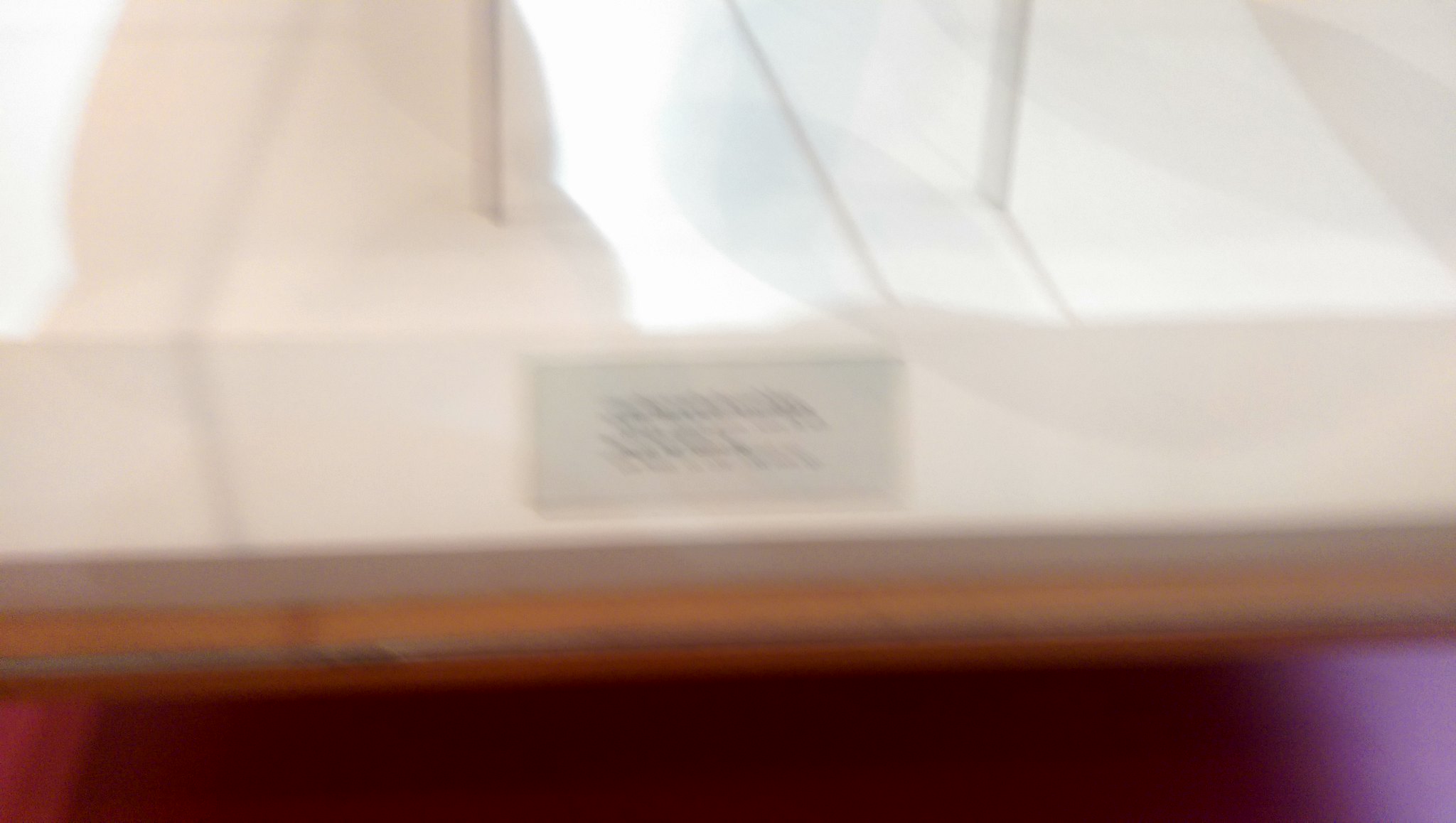On the side of the display, the lower section features a black area transitioning into a purple one towards the right. Above this section lies a large white rectangle, contrasting sharply with the darker tones below. Adjacently, there is a label that includes a small square and some textual information. The platform itself is a white square, and it appears to have an object protruding from its surface. A gray shadow is cast onto the platform, adding depth and dimension to the scene.